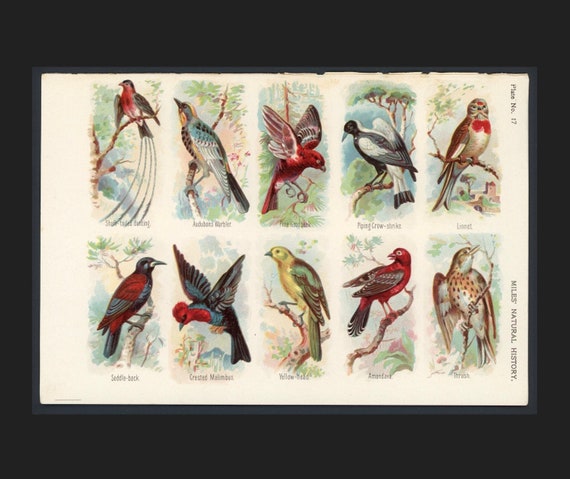This is an illustration of ten different kinds of birds, depicted in a watercolor or pen and ink style. The artwork is framed with a thick black frame and is set against a rectangular background. The birds are arranged in two rows, with five birds in the top row and five in the bottom row. Each bird is showcased in its own square frame and has its name labeled beneath it. The birds, varying from small to medium in size, display vibrant, tropical feathers. Two birds are predominantly red, while another two feature a mix of red, black, and blue. Among the collection, there is a bird that is yellow, green, and brown, and another that is brown with darker brown spots. One bird resembles a tan bird with a red chest, possibly an owl, while another striking bird looks like a bird of paradise. Noteworthy details include birds with long, elegant tails and others with shorter ones. Additionally, on the side of the illustration, there is a label that reads "Natural History."